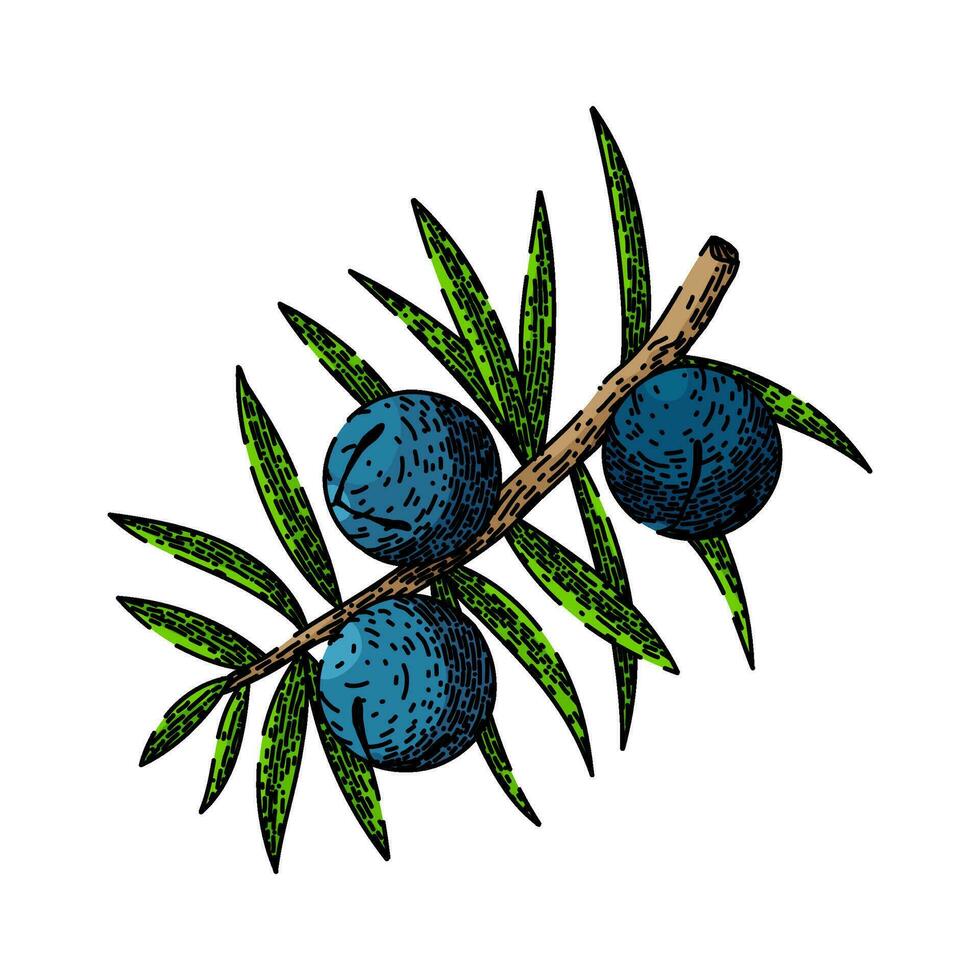This is a detailed color illustration depicting a small, brown branch adorned with numerous thin, deep green leaves, totaling eighteen. The branch features three small, spherical, deep-blue berries, resembling blueberries, positioned with one on the left of the branch and two on the right. The berries are marked with subtle white spots on two of their ends and delicate black lines. The arrangement shows one berry facing upwards, one facing downwards, and the third to the extreme right, also facing down. The illustration is set against a plain white background, emphasizing the botanical elements without any text or additional objects.